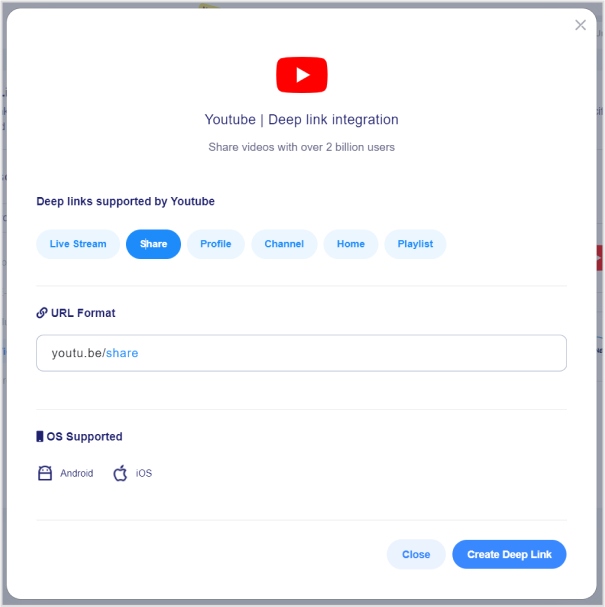The image showcases a landing page for YouTube's Deep Link Integration. Set against an all-white background, the page features the iconic red YouTube logo prominently at the top center. Just below the logo, the caption reads, "YouTube Deep Link Integration: Share videos with over 2 billion users." Following this, a subtitle states, "Deep Links supported by YouTube."

The page includes a row of functional buttons labeled: "Live Stream," "Share," "Profile," "Channel," "Home," and "Playlist." Directly below these buttons, there is a section titled "Link URL Format," accompanied by an address bar displaying "YouTube.be/share." Toward the bottom of the screen, the caption "OS Supported" is followed by the logos for Android and iOS, indicating platform compatibility. In the bottom-right corner, two buttons labeled "Close" and "Create Deep Link" are visible, presumably for navigation and link creation purposes.